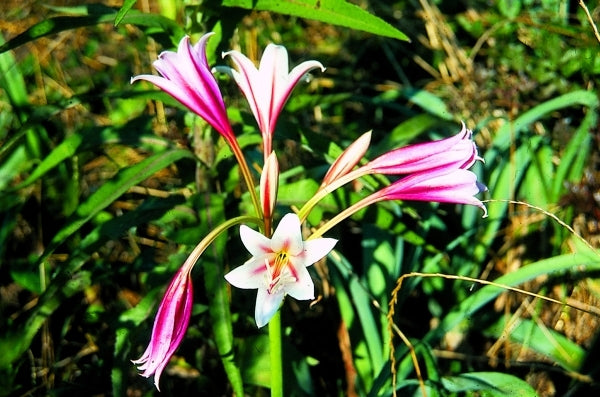This vibrant close-up image captures a cluster of blooming flowers, identified as types of lilies or irises, varying in shades of pink and purple. The focal point of the photograph is a central flower, partially opened, revealing delicate hues of whites and traces of yellow at its core. Surrounding the central bloom, multiple flowers, including a few fully open and others in various stages of unfolding, display a mesmerizing array of pinks and purples with edges that have a swirling appearance. The background is a sea of lush, green foliage comprised of long, grass-like leaves, punctuated by some brown leaves, creating a vivid contrast to the colorful blooms. The vibrant colors and intricate details of the flowers are sharply contrasted by the gradient shades of green leaves and stems, providing a serene backdrop to this exquisite natural scene.